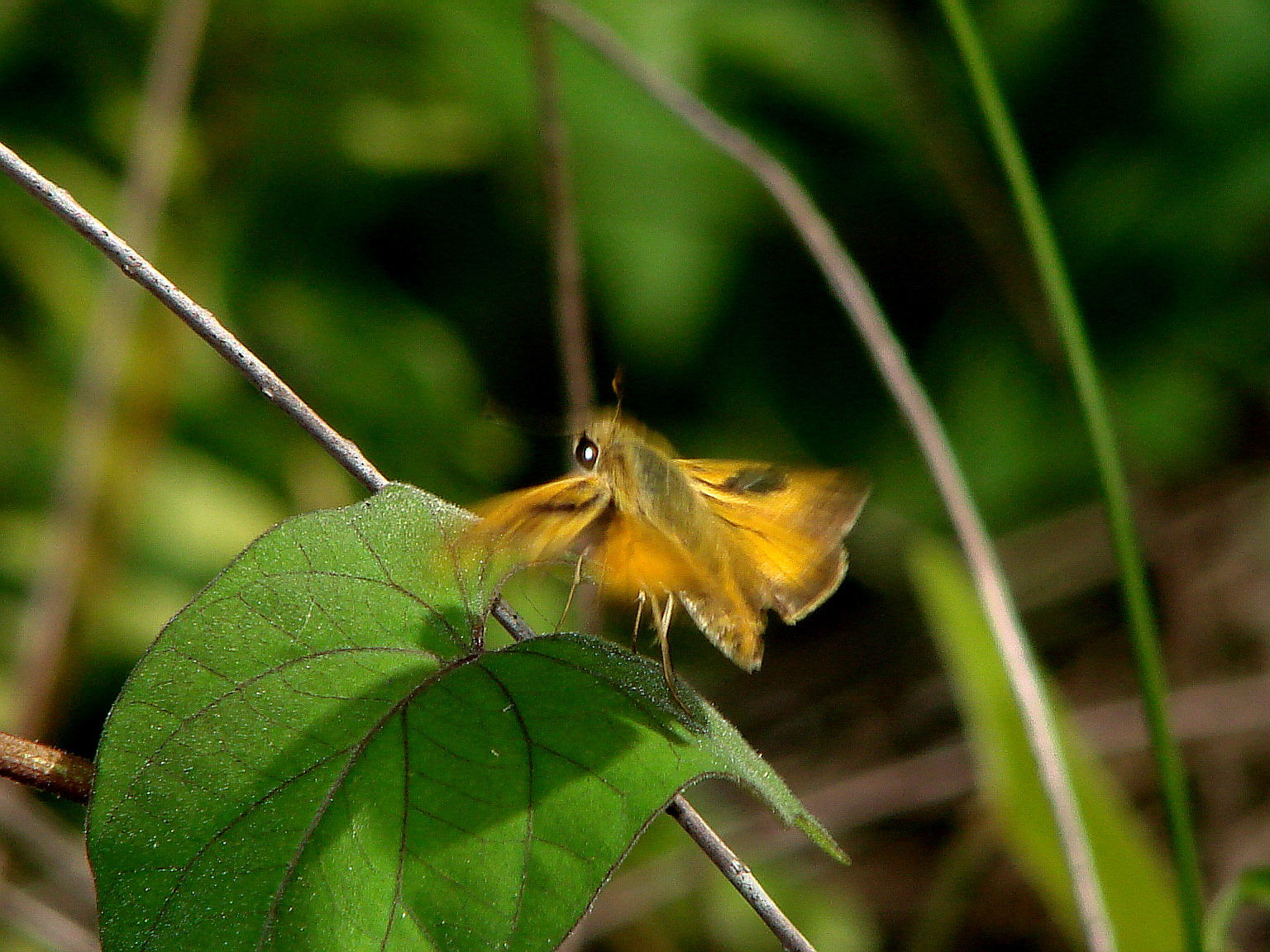A detailed close-up captures a yellowish-gold butterfly or moth with large black eyes and a black face marked by a white spot, landing on a large green leaf adorned with dark veins and specks of dew. The insect's furry body and wings, decorated with some green and black spots, appear hazy due to the rapid movement of its wings. A small twig extends diagonally from the midpoint of the right side towards the left corner, holding the leaf. Behind the sharp focus on the insect, leaf, and thin branches, the background features blurred greenery, adding depth to the vibrant and dynamic scene.